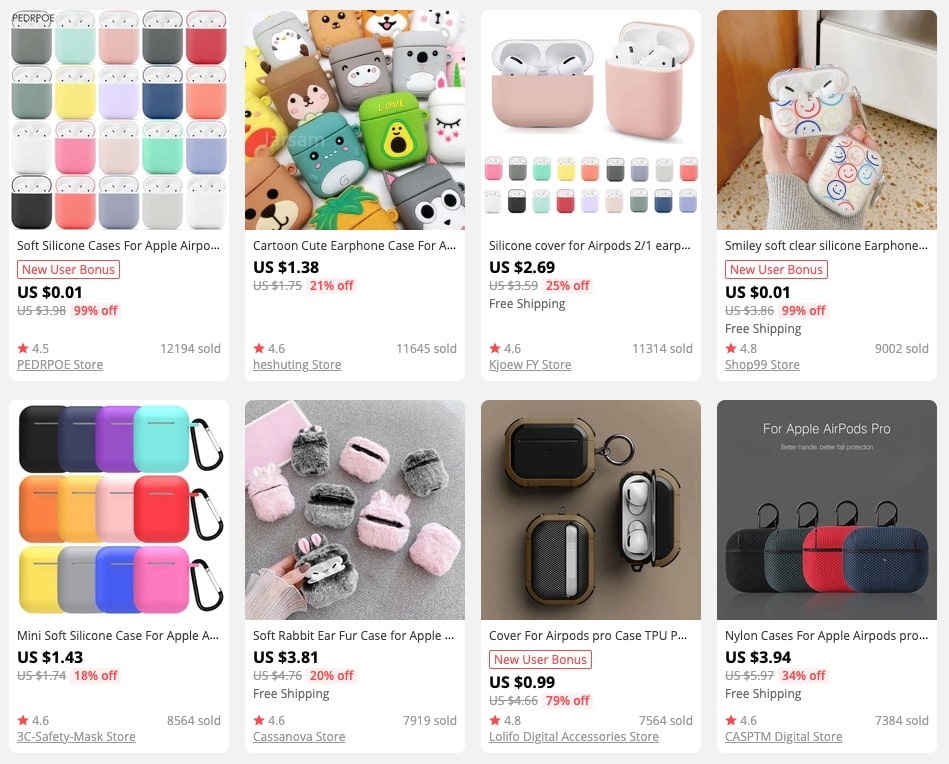This image is a rectangular screenshot from a shopping website, displaying a grid layout with two rows and four columns of AirPods cases. Each product listing within the grid follows a consistent structure: an image of the product at the top, followed by the product title, price, star rating, and the store name.

In the upper left-hand corner, the first product listing shows soft silicone cases for Apple AirPods under the watermark "P-E-D-R-P-O-E." The listing includes an image of several Apple AirPods cases arranged in a grid (five columns and four rows). It features a notable "New User Bonus" button, highlighting the product price as $0.01, which is 99% off the original price. This item has a 4.5-star rating and is sold by the P-E-D-R-P-O-E store, with 12,194 units sold.

The next product listing beside it is a cartoon cute earphone case marked with an "A-R-S-A-M" watermark on the image. The price is $1.38, offering a 20% discount, and is available from the HeShutting store.

The third listing in the sequence is for a silicone cover for AirPods priced at $2.69, which is 25% off the original price.

Completing the top row, the fourth product is a smiley soft clear silicone earphone case available for $0.01, representing a 99% discount.

This image captures a diverse range of AirPods cases with varying designs, discounts, and store ratings, providing a detailed snapshot of the available products on the shopping site.